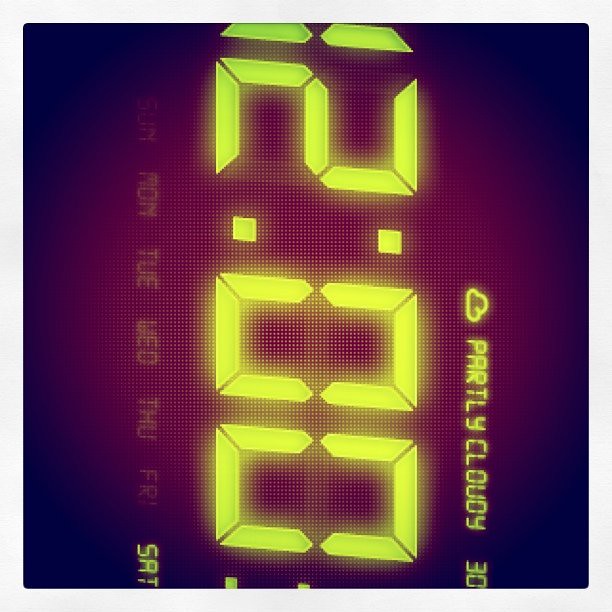This is a sideways photograph of a digital clock face, displayed in a vertical orientation. The close-up is sharp enough to reveal the individual pixels of the display. The clock shows the time as '12:00' in bright, fluorescent yellow digits. Above the time, there is a small cloud symbol with the text 'partly cloudy' and '30' underneath. The day 'Sat' (Saturday) is clearly illuminated, while other days of the week—'Sun', 'Mon', 'Tue', 'Wed', 'Thu', and 'Fri'—are dimly visible but not lit. The glowing yellow figures stand out against a dark, pixelated background, which has a reddish hue that intensifies around the illuminated elements and fades to black toward the edges. The image appears to be computer-generated, with a polished and detailed look that emphasizes the backlit effects and pixel detail.